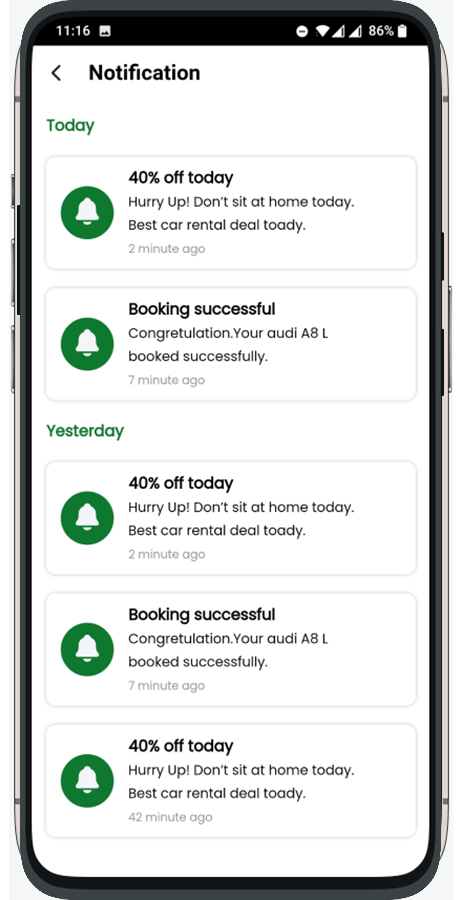This meticulously detailed mock-up showcases a realistic smartphone app interface. The phone, with elegantly curved corners, is set against a subtle light gray background that frames it neatly at each corner. The screen vividly displays the time, "11:16," positioned within a contrasting black bar at the top, accompanied by a photo icon in white. 

On the top right of the display, several status icons are visible, including a "Do Not Disturb" symbol, Wi-Fi connectivity, two signal strength indicators suggesting dual SIM card functionality, and a battery icon showing 6% remaining charge.

Dominating the main section of the screen is the app interface set against a clean white background. The heading reads "Notification," paired with a left-pointing arrow icon (<), followed by the green text "Today," delineating current notifications from previous ones. Beneath "Today," two concise notifications are displayed, while another section labeled "Yesterday" contains three additional notifications.

Each notification is marked by a green circle featuring a light gray bell icon, indicating activity. To the right of each bell icon, information is presented within a rectangular, shadowed box. For example, one notification reads: "40% off today, hurry up! Don't sit at home today. Best car rental deal today. 2 minutes ago," showcasing a timely and enticing offer. The remaining notifications follow a similar format, maintaining a cohesive and user-friendly design.